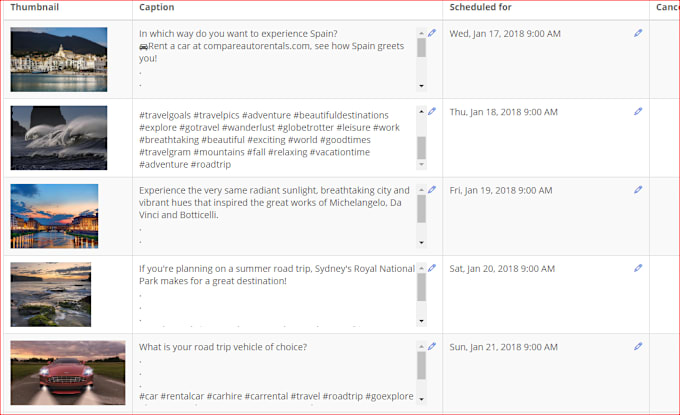Here is a detailed and cleaned-up caption for the provided image:

---

This image is a well-organized screenshot outlining a series of upcoming social media posts focused on travel, scheduled to be published at 9 a.m. on various dates in January 2018.

1. The first section features a thumbnail image representing a picturesque travel destination in Spain. The accompanying caption reads, "In which way do you want to experience Spain? Rent a car at compareautorentals.com. See how Spain greets you with a little slider bar so you can view more." This post is scheduled for Wednesday, January 17, 2018.

2. The second section showcases another thumbnail, along with a heavily hashtagged caption: "#travelgoals, #travelpics, #adventure, #beautifuldestinations, #explore, #gotravel, #wanderlust, #globetrotter, #leisure, #work, #breathtaking, #beautiful, #exciting, #world, #goodtimes, #travelgram, #mountains, #fall, #relaxing, #vacationtime, #adventure, #roadtrip." This post is scheduled for Thursday, January 18, 2018.

3. The third section describes an experience tied to a breathtaking visual of Italy: "Experience the very same radiant sunlight, breathtaking city, and vibrant hues that inspired the great works of Michelangelo, da Vinci, and Botticelli." This is set to be posted on Friday, January 19, 2018.

4. The fourth section presents a suggestion for a road trip destination: "If you're planning on a summer road trip, Sydney's Royal National Park makes for a great destination." This post is to be shared on Saturday, January 20, 2018.

5. The final section poses a question about travel preferences with vehicle keywords: "What is your road trip vehicle of choice?" It also includes hashtags: #car, #rentalcar, #carhire, #carrental, #travel, #roadtrip, #goexplore. This post is slated for Sunday, January 21, 2018.

---

Each post, complete with stunning thumbnail imagery and engaging captions, aims to inspire and inform travelers through a mix of practical information and evocative language.